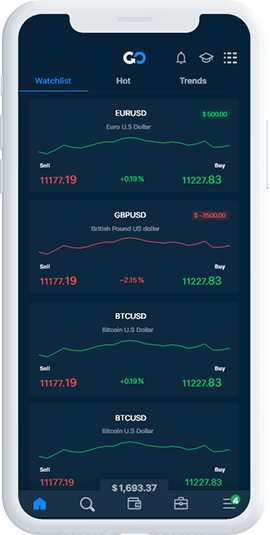The image depicts a silver phone against a navy blue background. On the left side of the phone, there are three buttons, and there is one button on the right side. At the top of the phone's screen, there is an infinity symbol with its left half in white and the right half in blue. Below the symbol, there is the outline of a white bell, followed by the outline of a white graduation cap. Additionally, there are three white circles, each containing two dashes aligned horizontally.

On the left side of the screen, in blue text, it states "Watchlist" positioned above what appears to be a money bill icon. Next to it in white text, it says "Hot and Trends."

Further down, there are four charts labeled with currency pairs. The first chart is labeled "USD," and the second one is "GBP/USD." The third chart shows "EUR/USD" for the Euro to U.S. Dollar pair, and the fourth one shows "BTC/USD" for Bitcoin to U.S. Dollar. Of these charts, the first, third, and fourth ones have green lines indicating a positive trend, while the second chart for the British Pound to U.S. Dollar shows a red line, indicating a negative trend. This suggests that while most currencies and assets are currently gaining value, the British Pound is experiencing a loss.